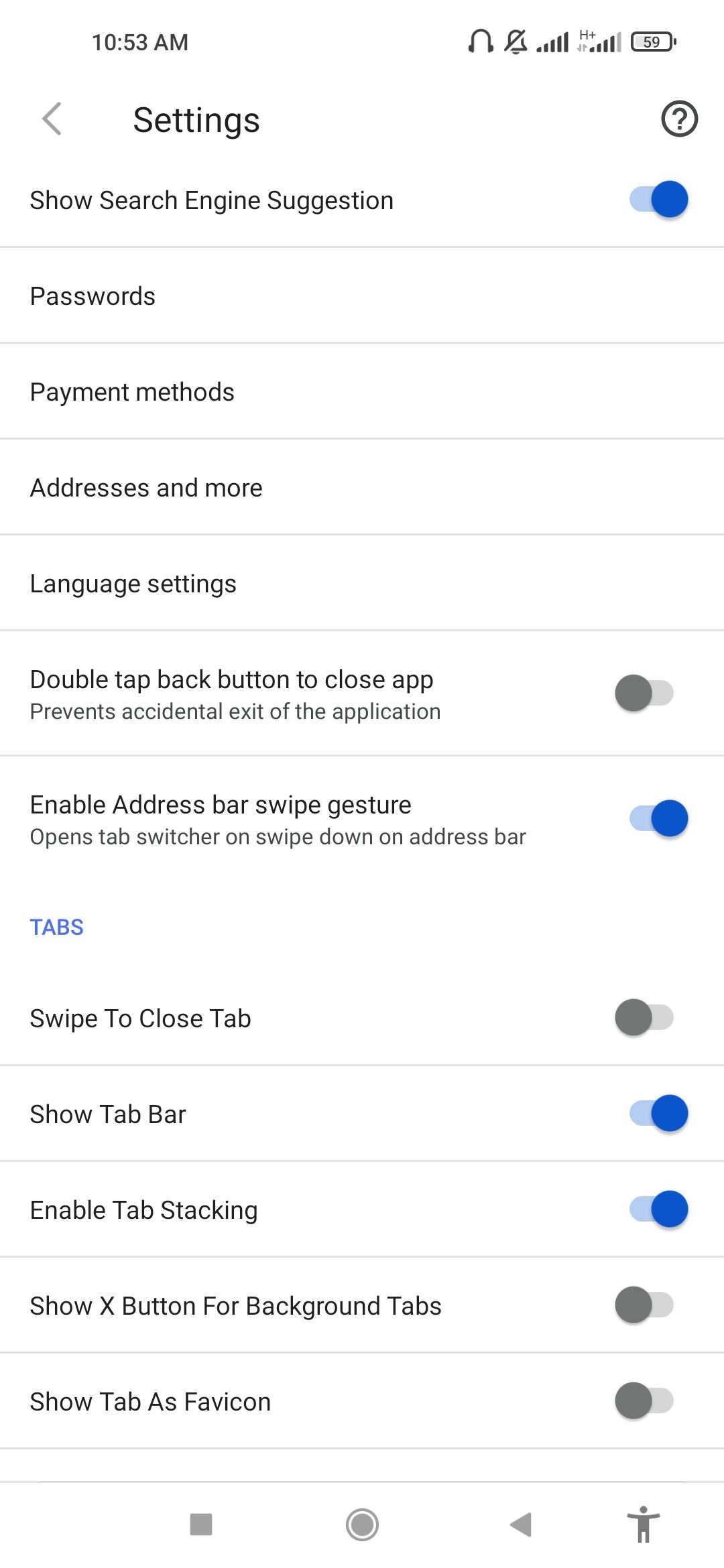The screenshot is vertically rectangular with a white background, captured from a cell phone under the "Settings" window. The image reveals the top left corner displaying the current time as 10:53 a.m. To the top right, various icons are visible. Centered on the left in all capital letters is the word "SETTINGS," followed by a vertical list of different options. 

- "Show search engine suggestion" has a toggle switch on the right, which is turned on.
- "Passwords"
- "Payment methods"
- "Addresses and more"
- "Language settings"
- "Double tap back button to close app," meant to prevent accidental exit, has an associated toggle that is turned off.
- "Enable address bar swipe gesture" with the toggle switch turned on.

Under the "Tabs" category:

- "Swipe to close tabs" has its toggle turned off.
- "Show tab bar" toggle is turned on.
- "Enable tab stacking" toggle is on.
- "Show X button for background tabs" toggle is off.
- "Show tab as favicon" toggle is turned off.